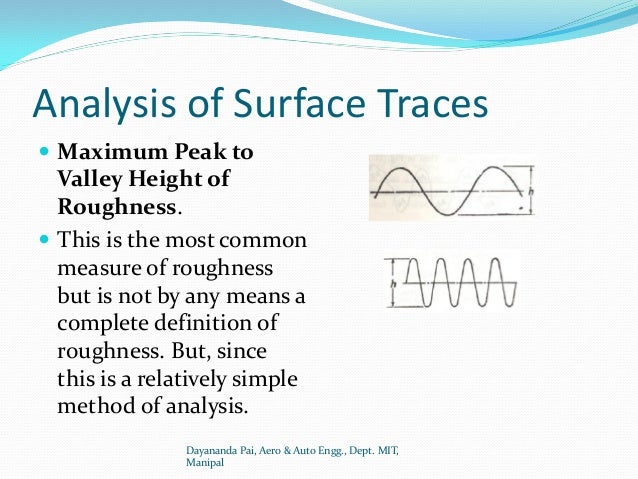The slide titled "Analysis of Surface Traces" features detailed information and visual aids focused on the measurement of surface roughness. At the top of the slide, a blue, wave-like design draws attention. Just below this, on the left, is the title in bold. Two main bullet points follow: the first in bold font stating "Maximum peak to valley height of roughness," and the second, not in bold, describing that while this is the most common measure of roughness, it is not a comprehensive definition; it is, however, favored for its simplicity in analysis.

Also on the slide are two graphics: the first, positioned centrally, shows a simple squiggly line, and directly beneath it is a more complex squiggly line with pronounced hills and valleys. The slide's background incorporates a palette of white, blue, black, and a hint of tan. At the very bottom, the text reads "Diamanda Pai, Arrow and Auto Engineering Department, MIT Manipal," providing information about the department and institution behind the analysis. This detailed descriptive layout appears to resemble content that might be found in an academic book or presentation.